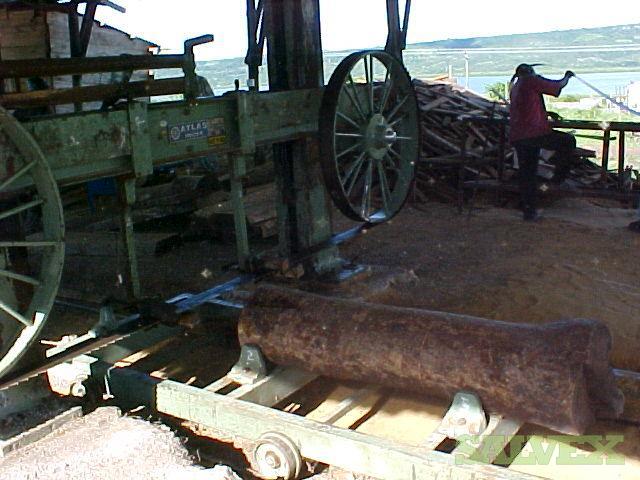The image captures an old, large, light green wood-processing machine with speckles of rust and white markings, prominently featuring the emblem "Atlas" in blue and white on its upper left corner. Central to the scene are two very large metal wheels with spokes that are integral to the machine's function. In the bottom right, a substantial log, about five to six feet long and a foot thick, rests on a conveyor roller, poised to be sliced by a significant blade. The machine is stationed on what appears to be the end of a railway track setup. To the left, a somewhat dilapidated structure with rusted metal girders and wooden beams can be seen, while in the middle-right foreground, a hefty cylindrical object lies on the rails between the large wheels. A pile of processed wooden planks is visible near a man wearing a red shirt and black pants, who is holding a straight, curved object and stands on dirt. In the distance, a sloping mountain, power lines, and a body of water stretch into the horizon, adding depth to the daytime outdoor industrial scene.